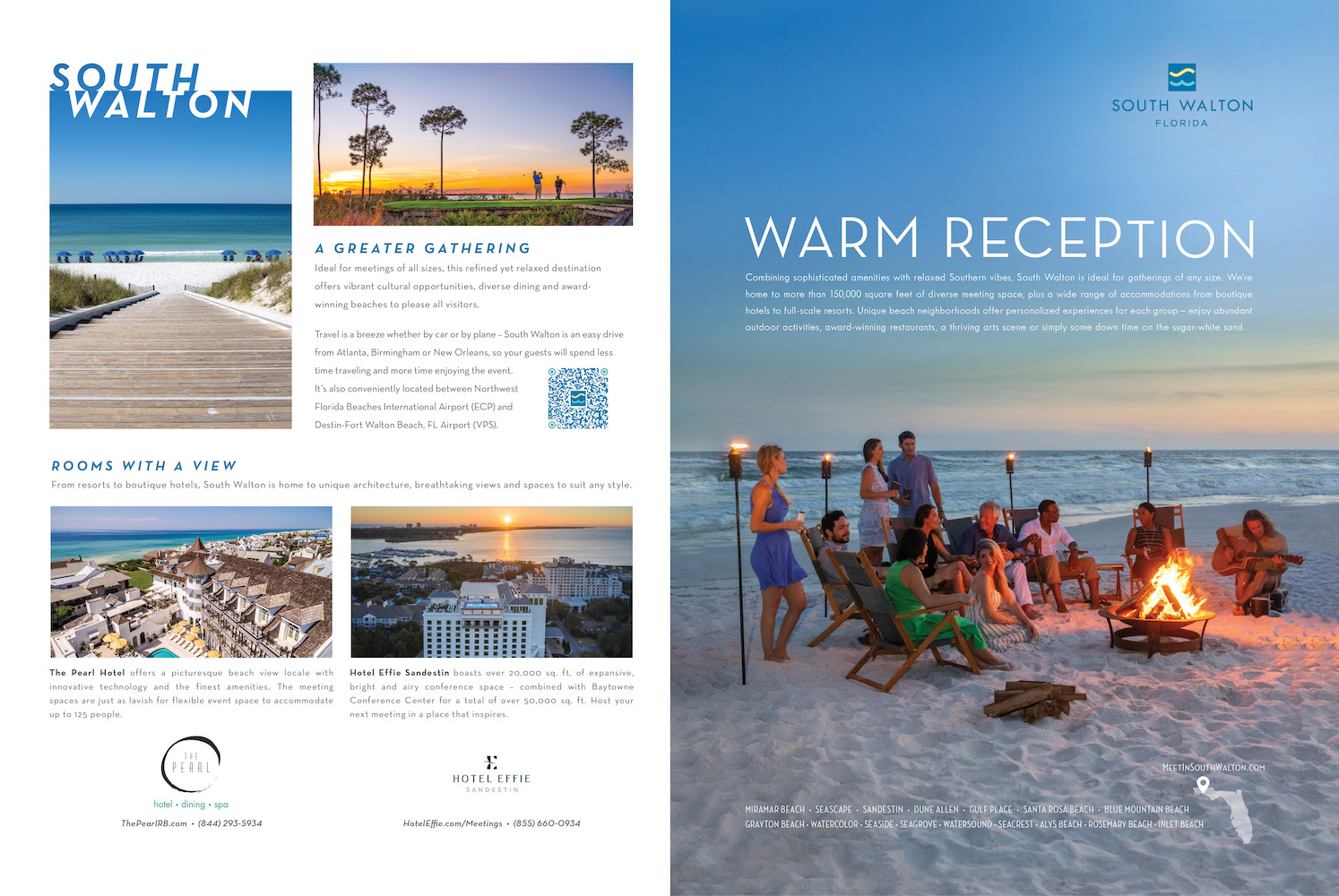The image appears to be a two-page spread from a magazine or pamphlet advertising a resort in South Walton, Florida. The background showcases a pristine beach with white sand and vibrant, almost translucent blue water. On the left page, bold text reads "South Walton," followed by "A Greater Gathering," and "Rooms with a View." Also on the left are four small images depicting various sunny spots around the resort, including The Pearl Hotel, although the finer text is difficult to decipher due to its size. The right page features a prominent picture labeled "A Warm Reception," capturing around 10 to 12 people, both men and women in their 30s, seated on wooden chairs around a campfire on the beach. One person is playing a guitar, and tiki torches add warmth to the scene. The group is dressed in vibrant colors such as blue, green, white, and red, and they appear to be enjoying a social, music-filled evening. A QR code is also present for additional information. The overall ambiance is tropical and inviting, emphasizing a sense of community and relaxation.